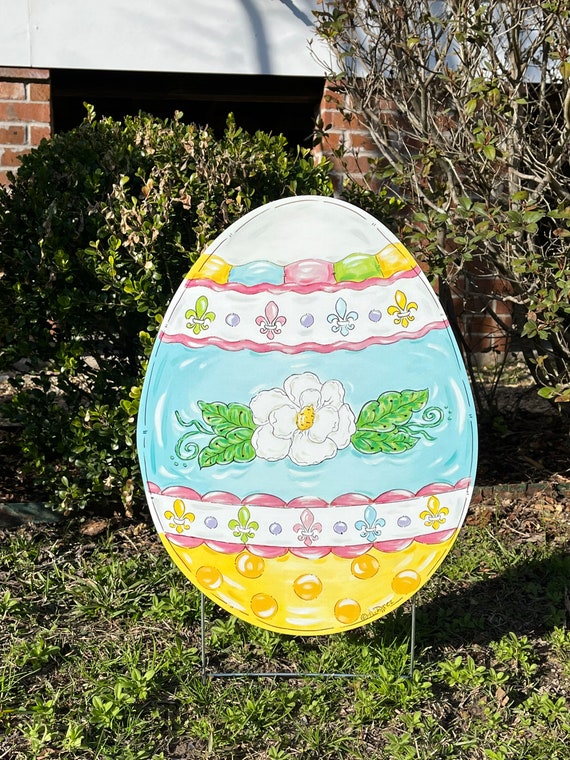This detailed image captures the front yard of a home, focusing on the central object, a large decorative Easter egg mounted on a metal stand. The egg is artfully cut out to resemble a real Easter egg and is adorned with colorful designs. At the very top of the egg, there is a white band followed by a ribbon-like variegated band featuring yellow, blue, pink, green, and yellow colors. Below this band, a white section showcases green, pink, blue, and yellow fleur-de-lis symbols. The egg's central band is a wide light blue stripe highlighting a white camellia flower with a yellow center, flanked by leaves and intricate curly-que tendrils. 

Lower on the egg, another white band replicates the fleur-de-lis pattern with the same colors as above. At the bottom, a yellow band is decorated with floating golden polka dots. The egg's vibrant colors include blue, yellow, purple, and green, and the design appears to have a watercolor finish.

In the background, part of the house is visible, displaying a combination of brick foundation and white siding. Surrounding the egg, there is a mix of green shrubbery and two trees, with the ground beneath it featuring patches of grass, dirt, and twigs. There is no text present in the image, allowing the colorful Easter egg and its detailed decorations to take center stage.